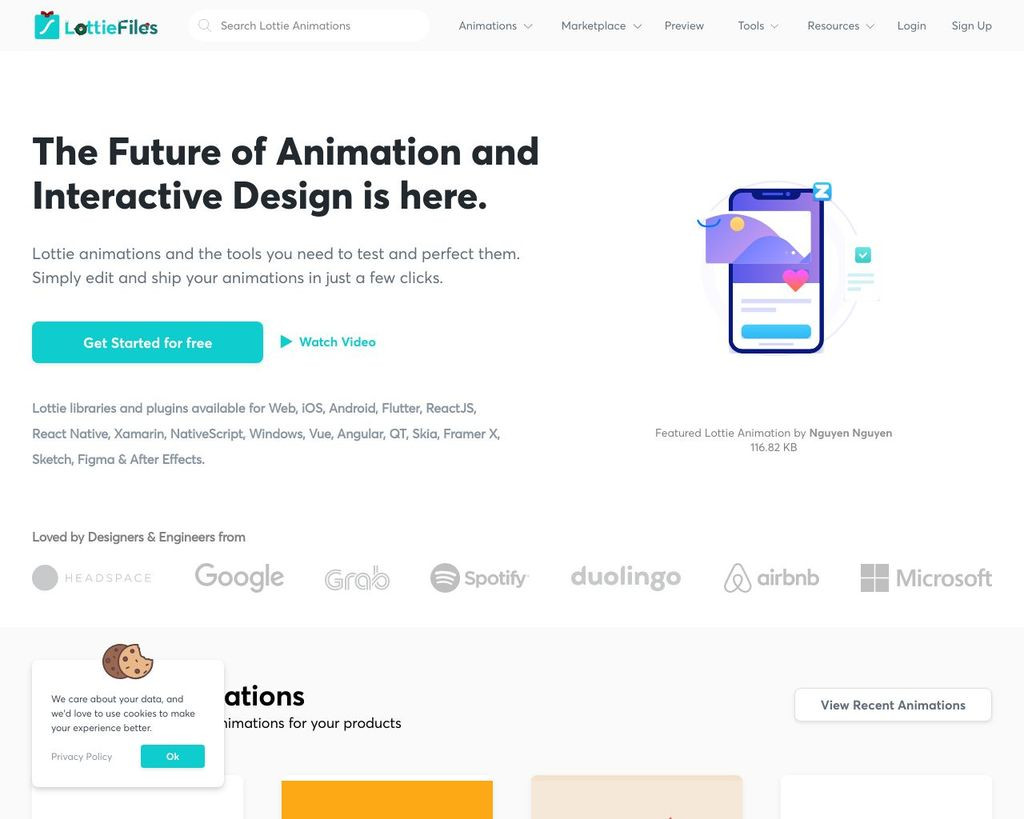Screenshot of the LottieFiles homepage: showcasing an array of features and tools for creating and editing animations. The webpage invites users to search for Lottie animations, explore the marketplace, preview tools, and access various resources. It prominently features call-to-action buttons for logging in, signing up, getting started for free, and watching an introductory video. A section highlights the compatibility with multiple platforms and proudly displays partnerships with prominent businesses such as Headspace, Google, Grab, Spotify, Duolingo, Airbnb, and Microsoft. The page also emphasizes the company's commitment to privacy. Towards the bottom, an orange button allows users to view recent animations, indicating the presence of a comprehensive Lottie library and plugins available for web sourcing.